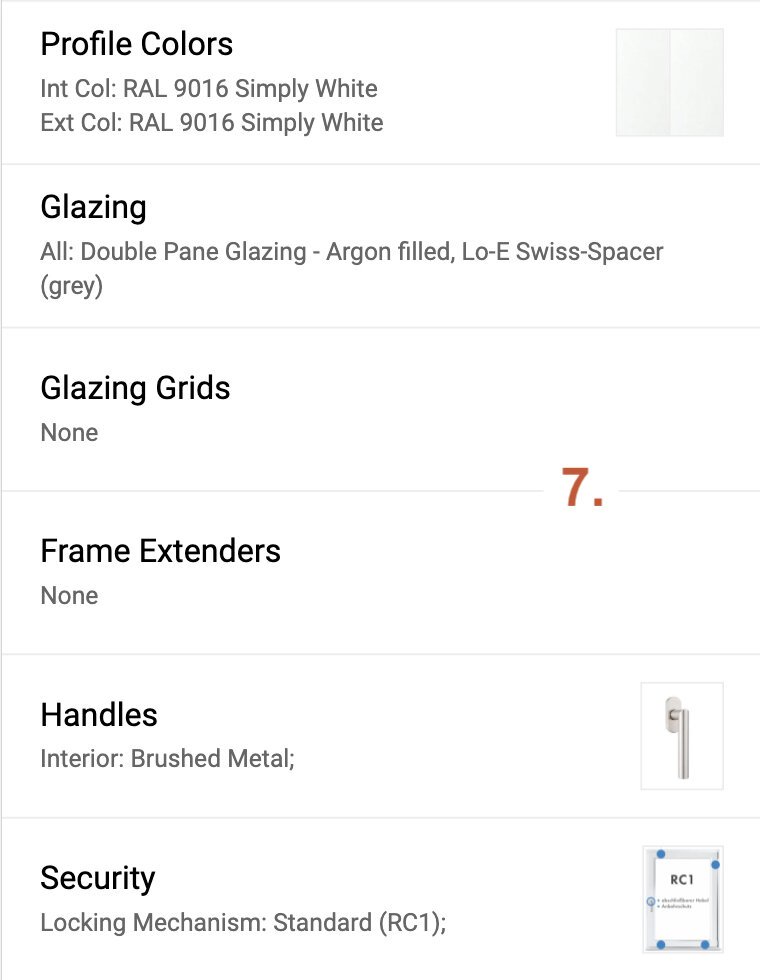The image features a meticulously detailed specification sheet against a white background, outlined in light gray. At the top of the sheet, the word "Profile Colors" is prominently displayed in black. Directly underneath, in gray font, it lists "IntCol: RAL 9016 Simply White" and "ExtCol: RAL 9016 Simply White," indicating both interior and exterior color codes.

Below these details, a gray-shaded box is depicted on each side of a fine gray dividing line, with the label "Glazing" in black. The glazing details, mentioned in gray, read "All double pane glazing - argon filled, low-e, Swiss spacer (gray)." 

Another fine gray line separates the next section, titled "Glazing Grids" in black, with "None" noted underneath in gray. Positioned about three-quarters to the right of the sheet, there is a red numeral "7" followed by a dot.

Continuing down, "Frame Extenders" is listed in black, with "None" stated in gray below it, separated by another fine gray line running across the page. 

Next, under the "Handles" section, written in black, the handle finish is described in gray as "Interior Brush Metal," accompanied by a small gray box displaying a depiction of a handle in a silver-like brushed metal finish.

The "Security" section follows, labeled in black with gray text beneath that reads "Locking Mechanism: Standard (RC1)." An outlined gray box is shown on the right, with a gray frame featuring blue dots at the top and bottom. Inside the box, "RC1" is clearly displayed, along with smaller black lettering within the interior of the box.